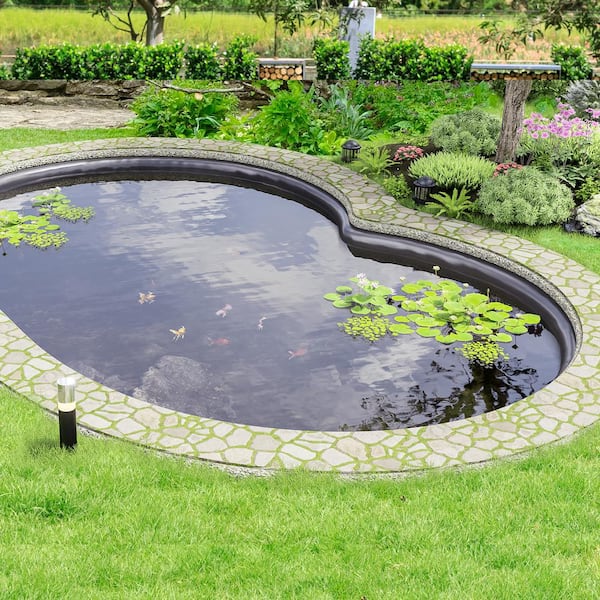This photograph showcases a tranquil garden setting featuring a man-made, kidney bean-shaped pond that has the appearance of a neglected pool. The water is dotted with clusters of lily pads, particularly in the bottom right and top left corners. At least six fish are visible swimming smoothly in the center of the pond. The pond is lined with small stones, beyond which lies a well-maintained landscape. The foreground is lush with green grass interspersed with flowering plants and mulchy areas, especially on the right side. A series of paved stones creates a walkway further past the pond, while the background reveals a variety of bushes, planters, a bird feeder, and a large field bordered by numerous trees. The scene is abundant with greenery, suggesting a serene and fertile environment.